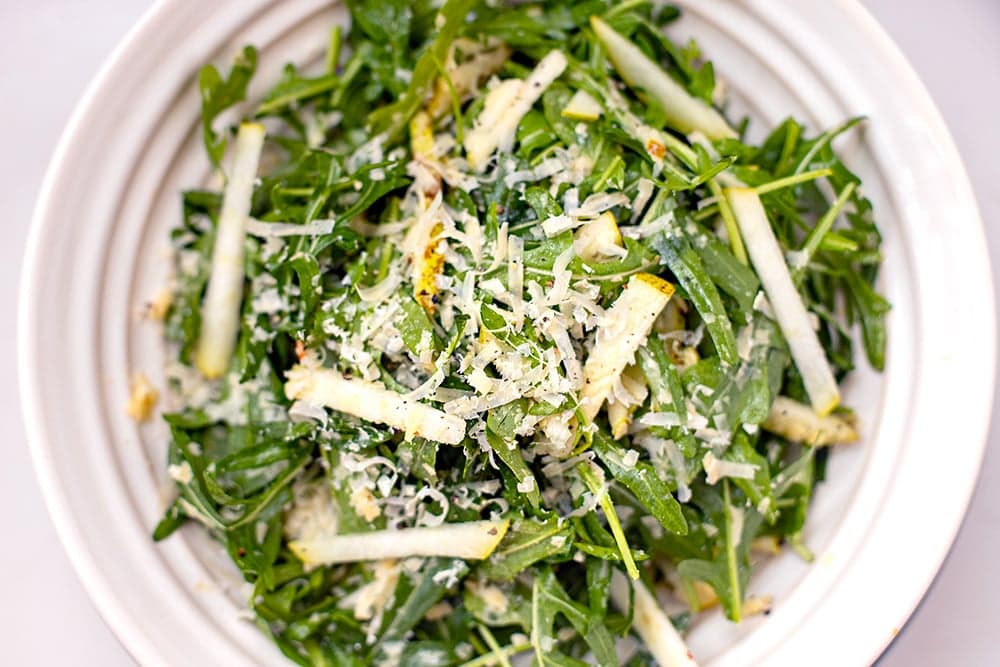An overhead view captures a bountiful salad in a plain white bowl with ridged edges, seated on a white surface tinged with pink. The lush salad is predominantly made up of very dark green leaves, likely kale, interspersed with white matchstick-like vegetable stems. Adding to the texture and flavor, there are noticeable shreds of white cheese liberally sprinkled, creating a snowy effect over the greens. Golden-tipped, cigarette-like shoots add a unique visual intrigue. The bowl is filled to the brim, giving the impression of abundant freshness. Small nuts are also sprinkled throughout, contributing to the variety of textures in this vibrant dish.